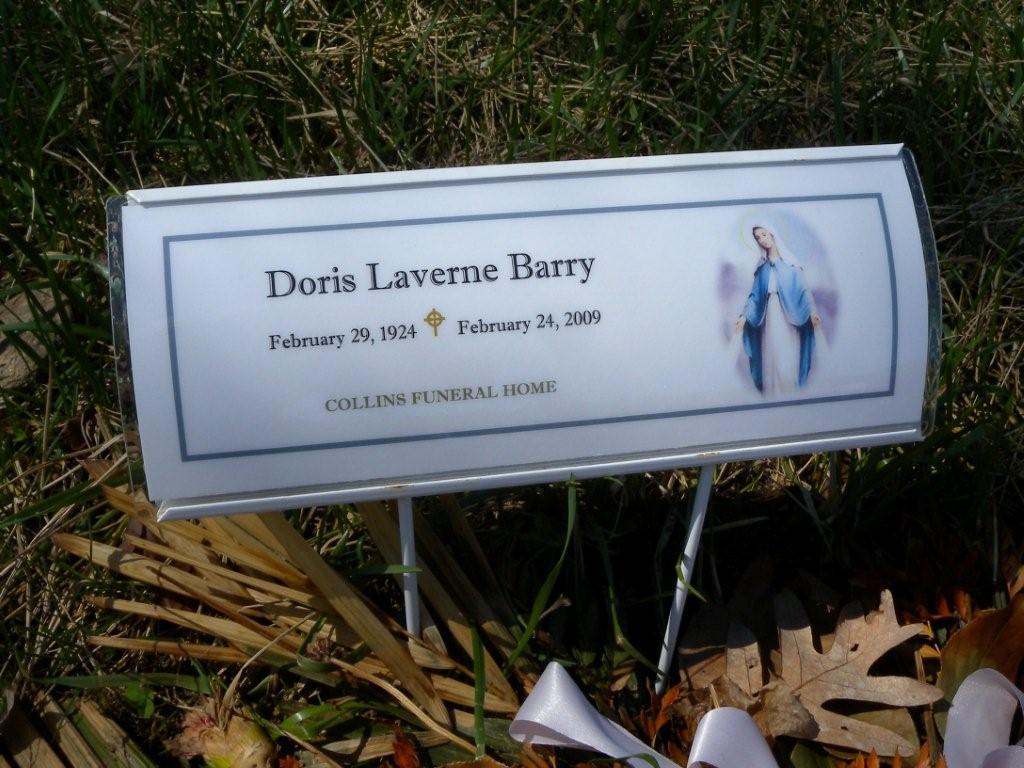This photograph captures a temporary grave marker for Doris Laverne Berry, who was born on February 29, 1924, and passed away on February 24, 2009. The white placard, encased in a silver-colored metal frame with a gray border, is staked into the green grass, amidst some fallen dead leaves and wilted flower bouquets. The placard prominently displays the name of the deceased, along with the dates of birth and death, and indicates the association with Collins Funeral Home. To the right of the text, there is an image of the Virgin Mary, adding a religious touch to this solemn marker. This temporary placard serves as a memorial until a permanent tombstone is installed.